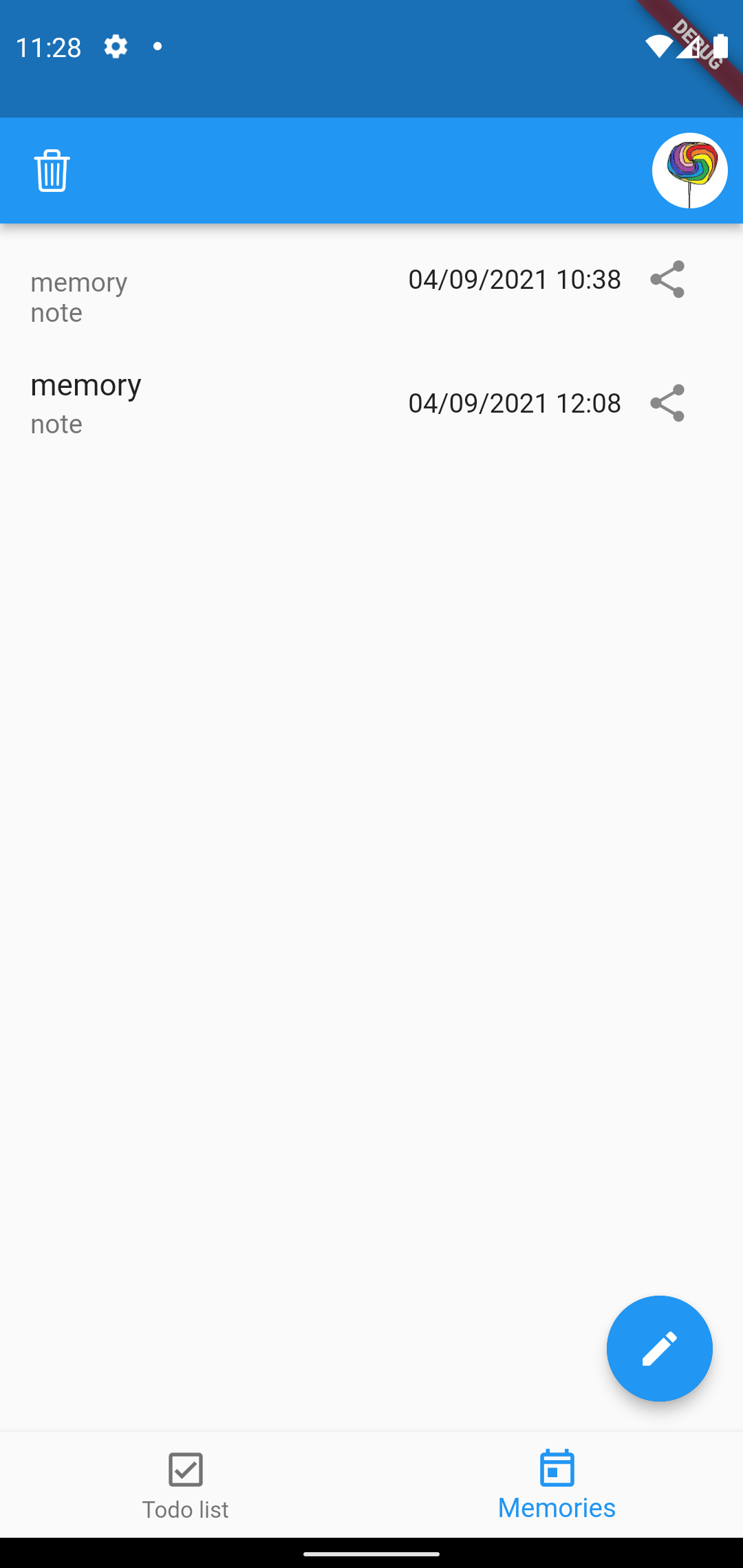This screenshot appears to be from an app or program interface on a phone. At the top, there is a blue, vertical rectangle featuring a settings button represented by a gear icon, the time [11:28], Wi-Fi connection status, battery level, and signal strength indicators. Below it is a lighter blue bar with a trash can icon on the left and a white circle on the right, containing a multicolored, abstract lollipop design composed of swirling lines and shapes.

Under this bar are two sections labeled as memory notes. The memory note at the top is grayed out and features a timestamp of [04-09-2021 10:38] alongside a share button that resembles a right-facing "V" shape. The second memory note, with a timestamp of [04-09-2021 12:08], is in a slightly larger font, indicating it is more recent. Both time entries are presented on a white background, with white and gray text.

At the bottom of the screen, there are navigation options labeled [2D List] and [Memories], and to the right, a blue circle with a white pen icon prompts users to add new entries.